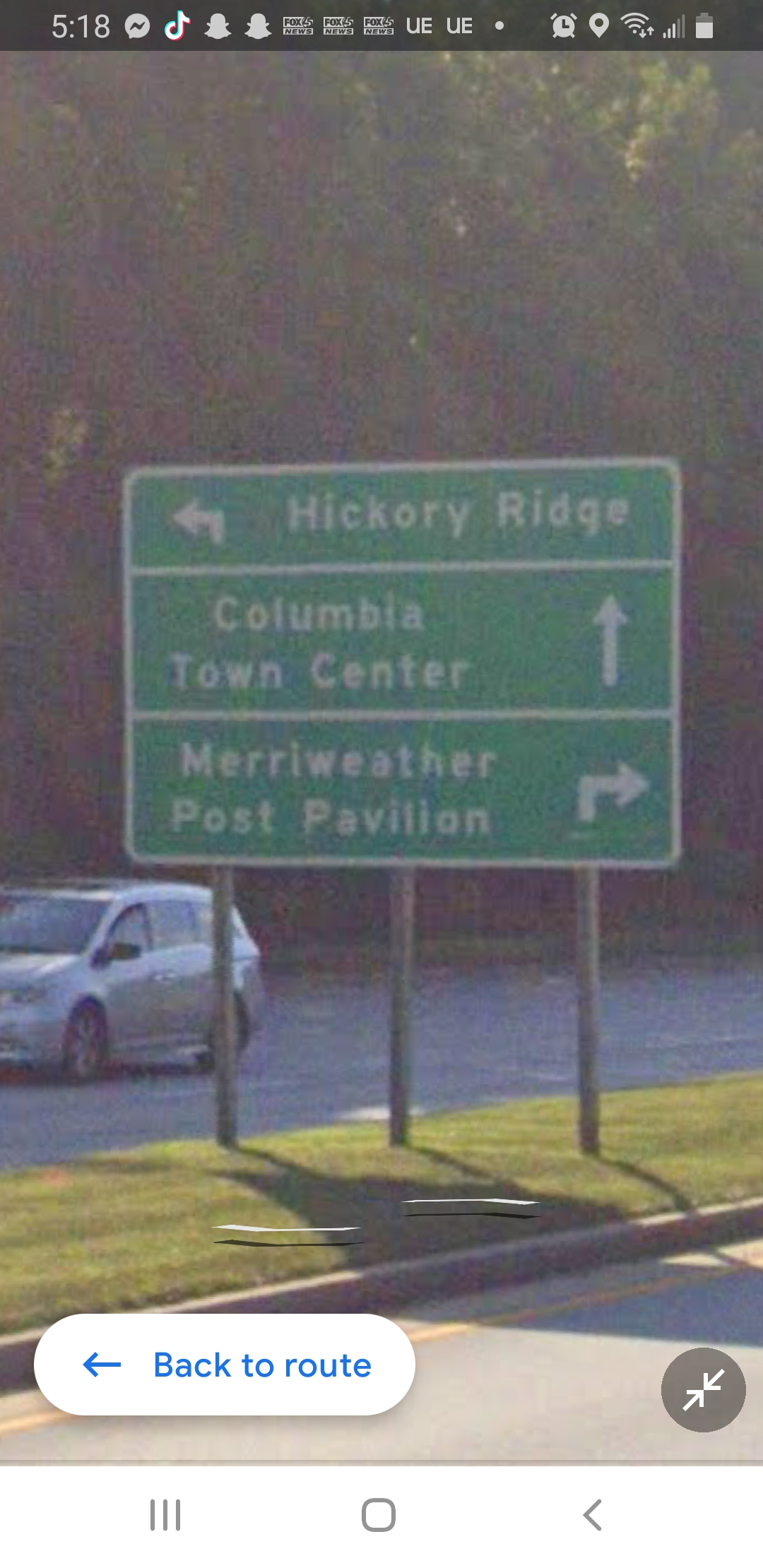This vertical, rectangular image appears to be a photograph taken on a smartphone, as indicated by the status bar at the top which displays the time (5:18), battery life, Wi-Fi signal, data coverage, alarm clock icon, and logos for TikTok and Messenger.

The image showcases a green street sign situated on a green inlet or nature strip that separates two roads. The rectangular, horizontal sign is divided into three sections by white horizontal lines. The top section features the text "Hickory Ridge" with a bold, left-pointing arrow. The middle section reads "Columbia Town Center," with a straightforward, upward-pointing arrow. The bottom section displays "Meriwether Post Pavilion" with a horizontal, right-pointing arrow. The sign is supported by three metal posts.

In the background, a light-colored car is seen driving along the left side of the image, and there are numerous trees providing a natural backdrop. At the bottom left corner of the image, a white oval button with bright blue lettering reads "Back to Route" and includes a left-pointing arrow. To the right of this button, there is a gray circle with two diagonal arrows facing each other, indicating zoom options.

Overall, this detailed image encapsulates a green street sign directing to different locations, set against a backdrop of trees and roads, emphasizing the natural and navigational elements.